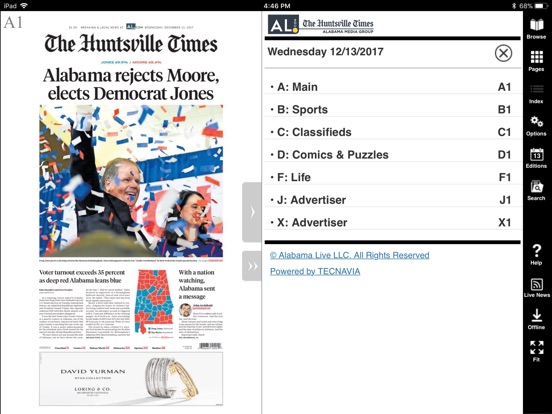Screenshot of an iPad displaying a digital newspaper. 

At the top, a thin black bar spans the width of the screen, indicating the device is an iPad. The status bar shows a full-strength Wi-Fi signal, the time "4:46 PM," active Bluetooth, 68% battery, and the battery icon. Along the right-hand side of the screen, another thin black bar vertically lists icons labeled Browse, Pages, Option, a partially readable icon, Search, Help (indicated by a question mark), Live News, Download Offline, and Fit (denoted by four arrows).

The central content features a digital edition of the "Huntsville Times" in old English-style script. The prominent headline reads: "Alabama Rejects More, Elects Democrat Jones," accompanied by a photograph of Democrat Jones, hand raised, amidst falling confetti. A woman is visible in the bottom-right corner of the photo.

Below the headline, an article reports on voter turnout exceeding 35% in Alabama, traditionally a deep-red state, hinting at a political shift. A map of Alabama displays red and blue counties. Another article, "With Nation Watching, Alabama Sent a Message," discusses the broader implications of the election.

At the bottom of the page, there is an advertisement for David Yurman jewelry featuring images of silver and gold earrings.